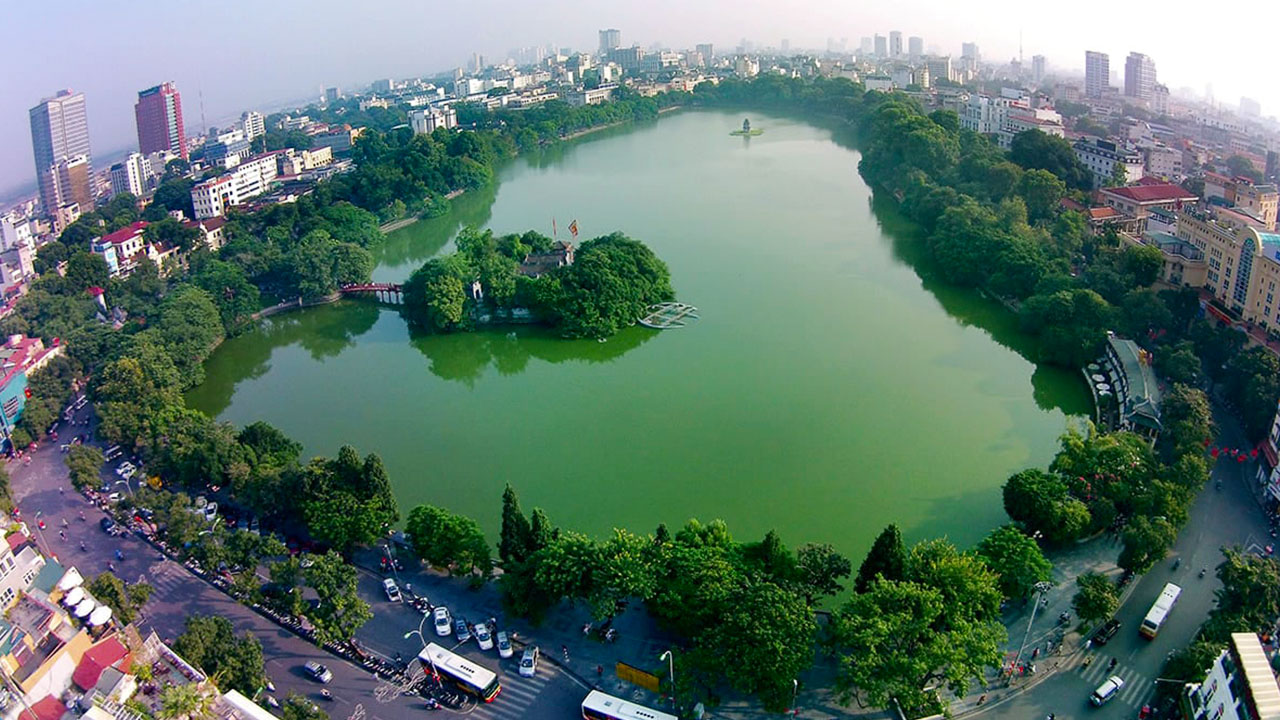This is an aerial photograph of a large, almost heart-shaped lake situated at the center of a bustling city. The lake's water is a striking emerald green, possibly due to algae, and is encircled by a dense canopy of healthy, deep green trees. To the left and right of the lake, roads encase it, with multiple buses and cars navigating them. On the bottom left corner, a small parking lot can be seen, receiving several buses, while the lake’s right side houses a slightly curved building with outdoor tables. In the background, a diverse skyline of tall skyscrapers and shorter buildings, some white with red roofs and others yellow, dominate the horizon under a hazy, polluted sky. 

A blacktop street wraps around the lake, busy with vehicles and people, some walking and others on bikes. A significant feature of the lake is a pier that extends halfway into the water, leading to a small island with a building and what appears to be a boat dock. The island hosts another structure, possibly for events, indicated by a visible flag. Further enhancing the picturesque quality of the scene, a small bridge connects the pier to the island, completing the near heart-shaped form of the lake.